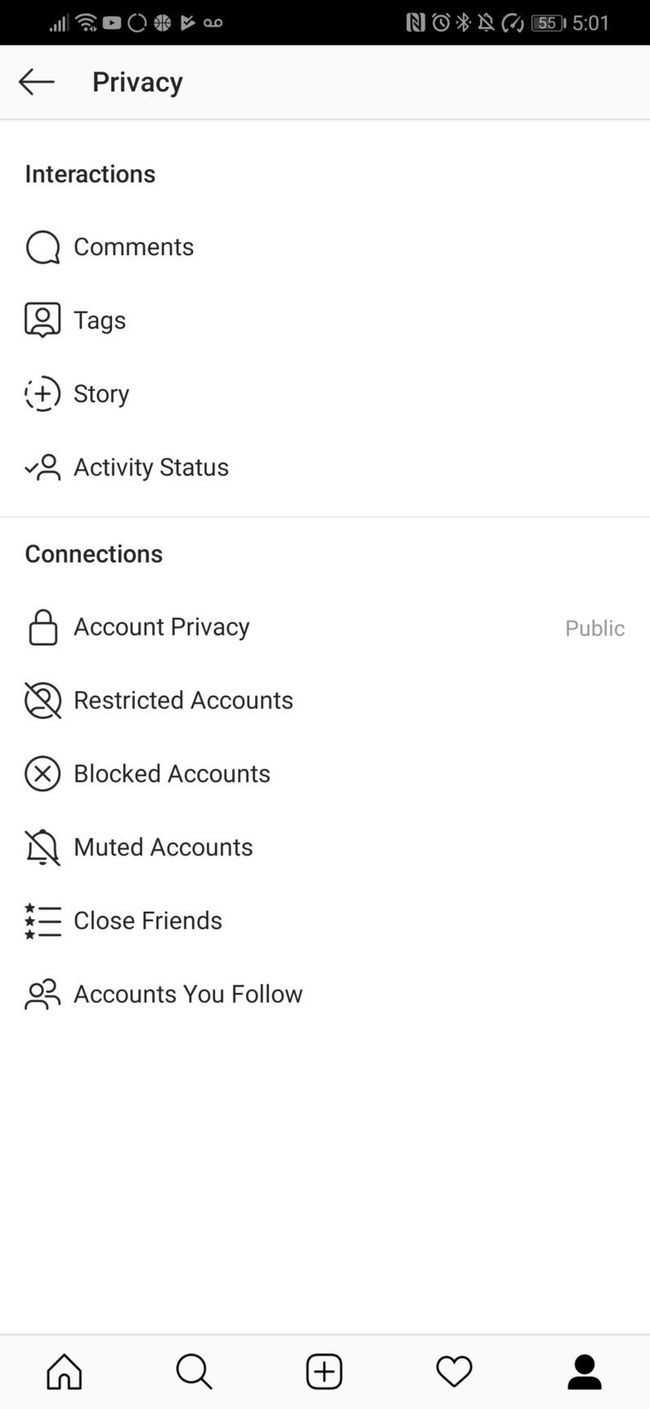The image displays the Privacy Settings page of the Instagram app. At the top of the screen, there is a header labeled "Privacy" accompanied by a left-facing arrow icon, allowing for backward navigation. Directly beneath this header, the main menu items are listed in a vertical arrangement, presenting options such as Interactions, Comments, Tags, Story, Activity Status, Connections, Account Privacy, Restricted Accounts, Blocked Accounts, Muted Accounts, Close Friends, and Accounts You Follow.

The background of the page is a pristine white, creating a clean and uncluttered appearance. At the very bottom of the screen are five primary navigation icons: a Home icon, a Search icon, a Plus (+) icon for new posts, a Heart icon for activity or likes, and a Profile icon for accessing the user's account.

The top section of the image features a black bar, which houses various status indicators including a Wi-Fi icon, the YouTube icon, a Clock icon, Bluetooth icon, an Alarm icon, and the current time.

Overall, the layout is user-friendly and intuitively designed, allowing for seamless navigation through privacy settings on the Instagram app.